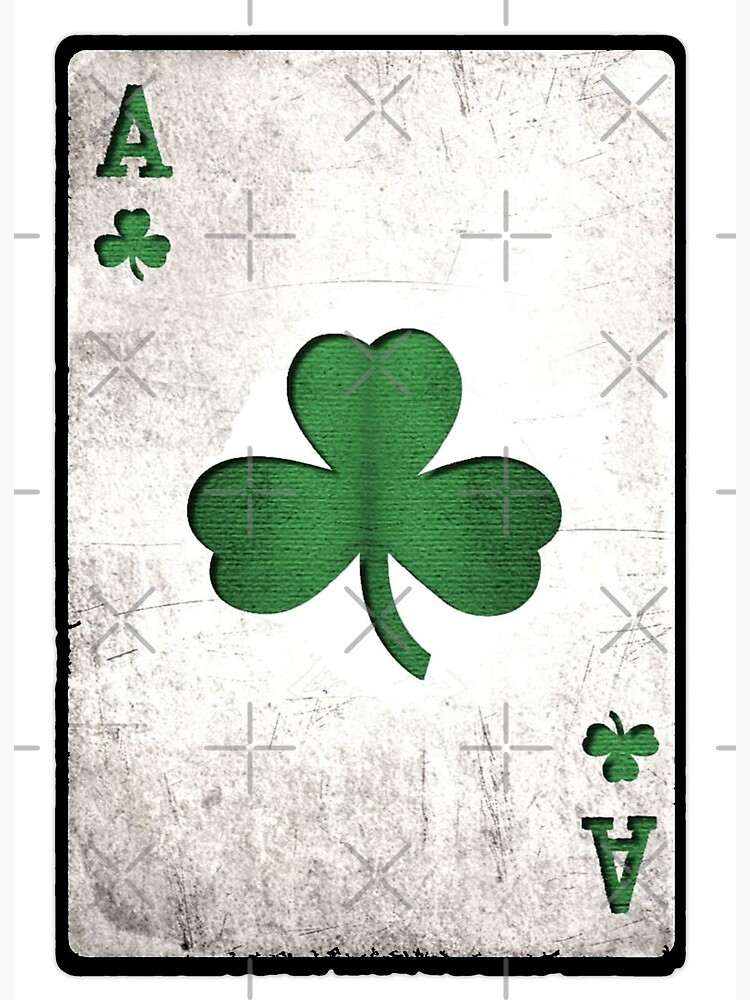This image features a playing card, specifically the ace of clubs. Notably, the card deviates from the traditional black-and-white design, being predominantly rendered in green. The card's white surface appears significantly dirty and scuffed, suggesting it had been dropped and trampled on. Both the top left and bottom right corners of the card are marked with a green 'A,' indicating its ace status, with smaller green three-leaf clovers situated beneath each 'A.' At the center of the card is a larger green three-leaf clover. A black frame outlines the card, further emphasizing its worn and grimy appearance. The overall color palette includes hues of emerald green, black, gray, off-white, and white.